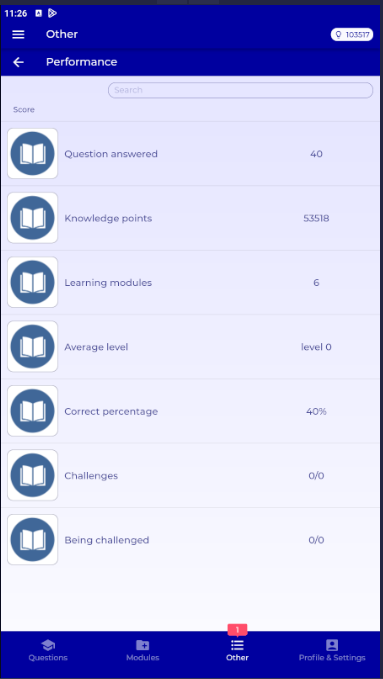This image appears to be a screenshot taken from a mobile device, either a phone or a tablet. It's a capture of an online learning or testing application, where the screenshot seems incomplete as parts of the edges are missing. 

At the top, there's a visible time stamp showing "11:26," along with a Google Play notification. The top segment showcases a blue bar with a context menu on the left side and another option, possibly a settings icon, on the far right. Below this top bar, there is another blue bar labeled "Performance," featuring a back arrow to its left and a small, gray-white search bar below it.

The application section under these bars contains several statistics and icons. Each icon appears as an open book with a blue circle behind it. Accompanying text details the user's performance metrics:
- Questions Answered: 40
- Knowledge Points: 5318
- Learning Modules: 6
- Average Level: 0
- Correct Percentage: 40%
- Challenges Completed: 0/0 

Additionally, there's a navigation menu at the bottom of the screen with tabs labeled "Questions," "Modules," "Other," "Profile," and "Settings." Notably, the "Other" tab has a red notification box with the number "1" in it.

From the visible performance metrics and layout, this application seems to function as an online testing or learning platform. The statistics suggest that the user has not performed well, as indicated by a low average level and a lack of completed challenges.